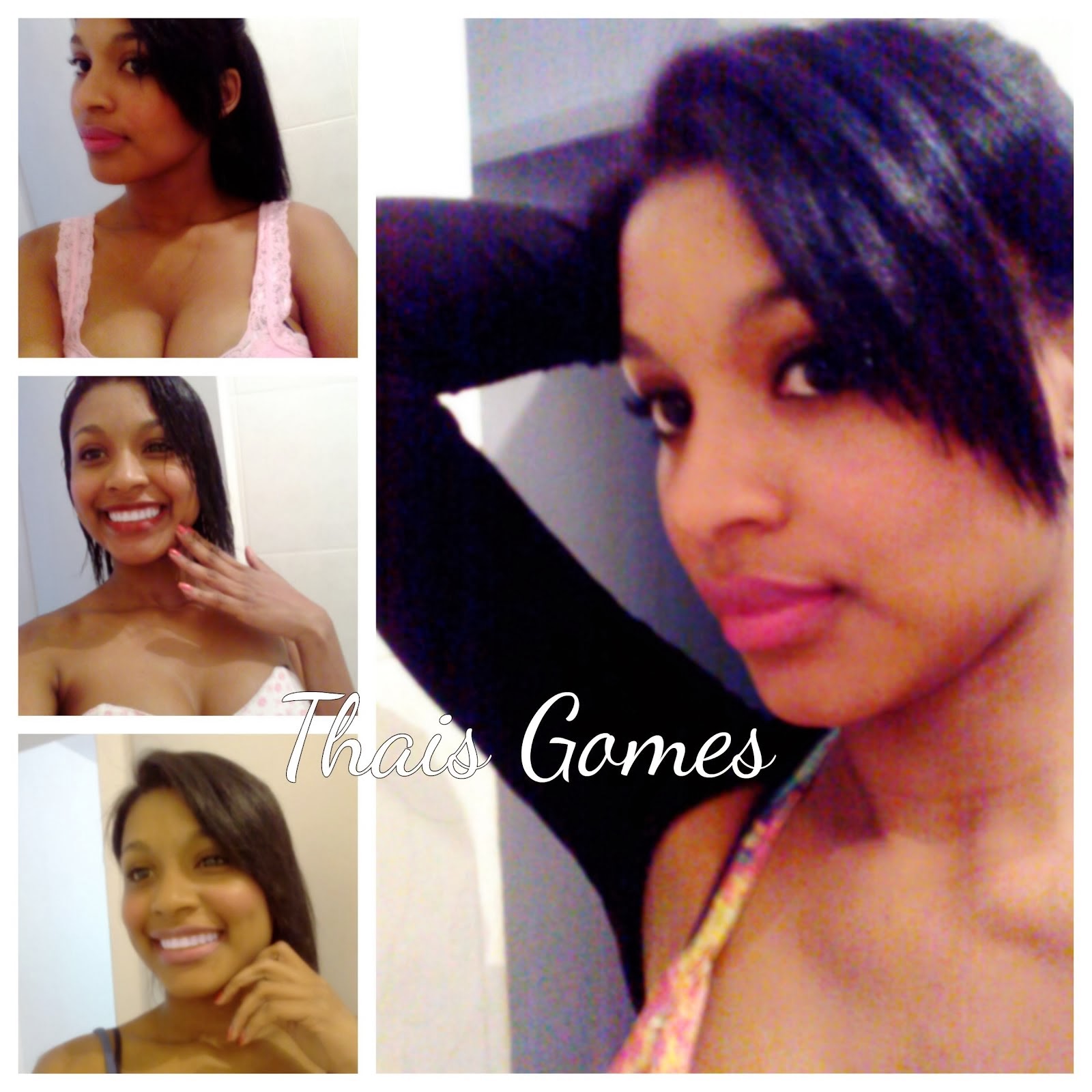The image features a collage of four photos of a woman, likely Asian, with dark hair. On the left side, three smaller photos are arranged vertically. In the top-left photo, she is wearing a pink tank top and looking to the right, her hair reaching her shoulders. Below this, the middle-left photo shows her smiling with wet hair, her left hand touching her cheek, dressed in a white tank top with dots. The bottom-left photo captures her again with her left hand on her chin, smiling brightly and wearing a blue tank top with a visible black strap. The photos primarily show her from the chest up. On the right side, a larger image of her displays her smirking slightly with pink lipstick on, her right arm behind her head, and a black sleeve visible. Across the middle of the image, the text reads "Thias Gomes" in white. The collage employs a scattered arrangement typical of social media sharing, utilizing colors like black, gray, white, pink, and hints of red, brown, and olive.